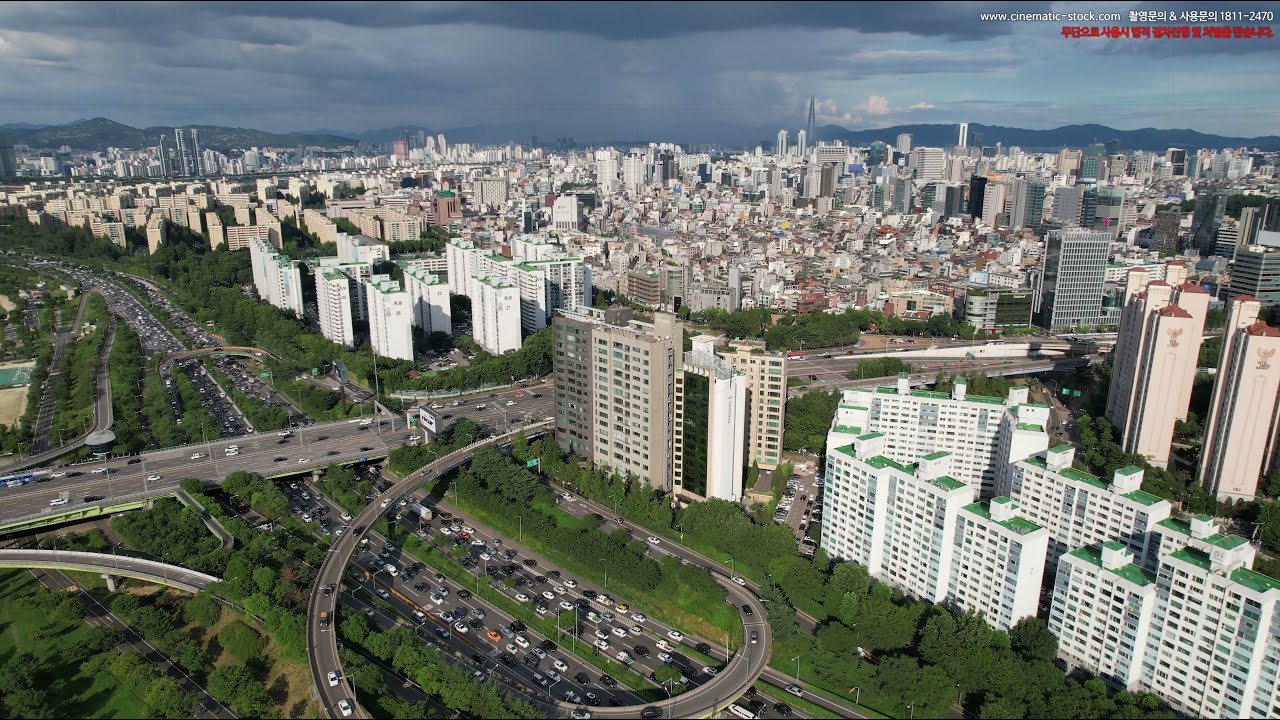The overhead view captures a bustling city teeming with life and movement. Dominating the bottom left corner, an interstate brimming with cars snakes from the upper left towards the center, featuring a roundabout and a turnpike diverting into the city on the right. The cityscape is densely packed with towering white buildings adorned with green rooftops, standing prominently in the forefront. These numerous identical structures are interspersed with light and dark brown buildings situated near the center. The city's expansive skyline reveals additional skyscrapers in the distance, framing a landscape bustling with activity. Shorter buildings dot the middle ground, surrounded by patches of green trees and grassy areas interspersed among the urban jungle. The horizon is marked by a distant row of mountains, shrouded in rain from dark, looming clouds. A website URL, www.cinematicstock.com, along with Asian characters and the numbers 1811-2470, is inscribed in white in the upper right corner, with further text in red characters beneath it, contrasting against the blue and gray cloud-filled sky. The scene is a vibrant, chaotic snapshot of city life, capturing the essence of a metropolitan hub in relentless motion.